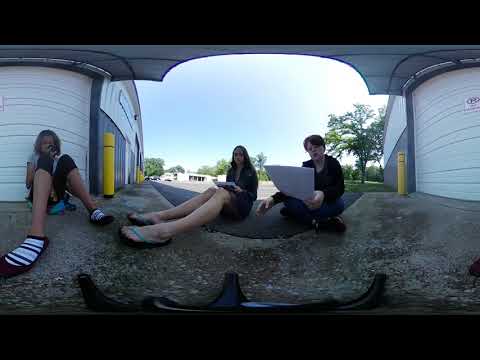The image features a horizontally aligned rectangular picture bordered by solid black lines at the top and bottom, capturing three individuals seated on a cement ground between two buildings under a partly cloudy sky. Both buildings have cylindrical white structures with yellow poles outside and garage doors visible on their sides. The setting includes some trees and a lawn, indicating a daytime outdoor scene.

At the center of the image, three teenagers are seated:

1. On the left, a person wearing black capris (or dark tights) and a white (or beige) shirt intently looks at a cell phone. They have short hair and are wearing sandals with striped socks.

2. The middle individual, a young woman with long brown hair, is dressed in a dark-colored shirt or coat, shorts, and flip-flops (or possibly pants and sandals). She is holding papers or a folder and looking directly at the camera.

3. To the right, another young person with short hair is seated cross-legged. They wear jeans and a dark shirt, holding a stack of papers that they appear to be reading from.

The wide-angle shot slightly distorts the scene to encompass the entire setting and the interaction among the three friends.